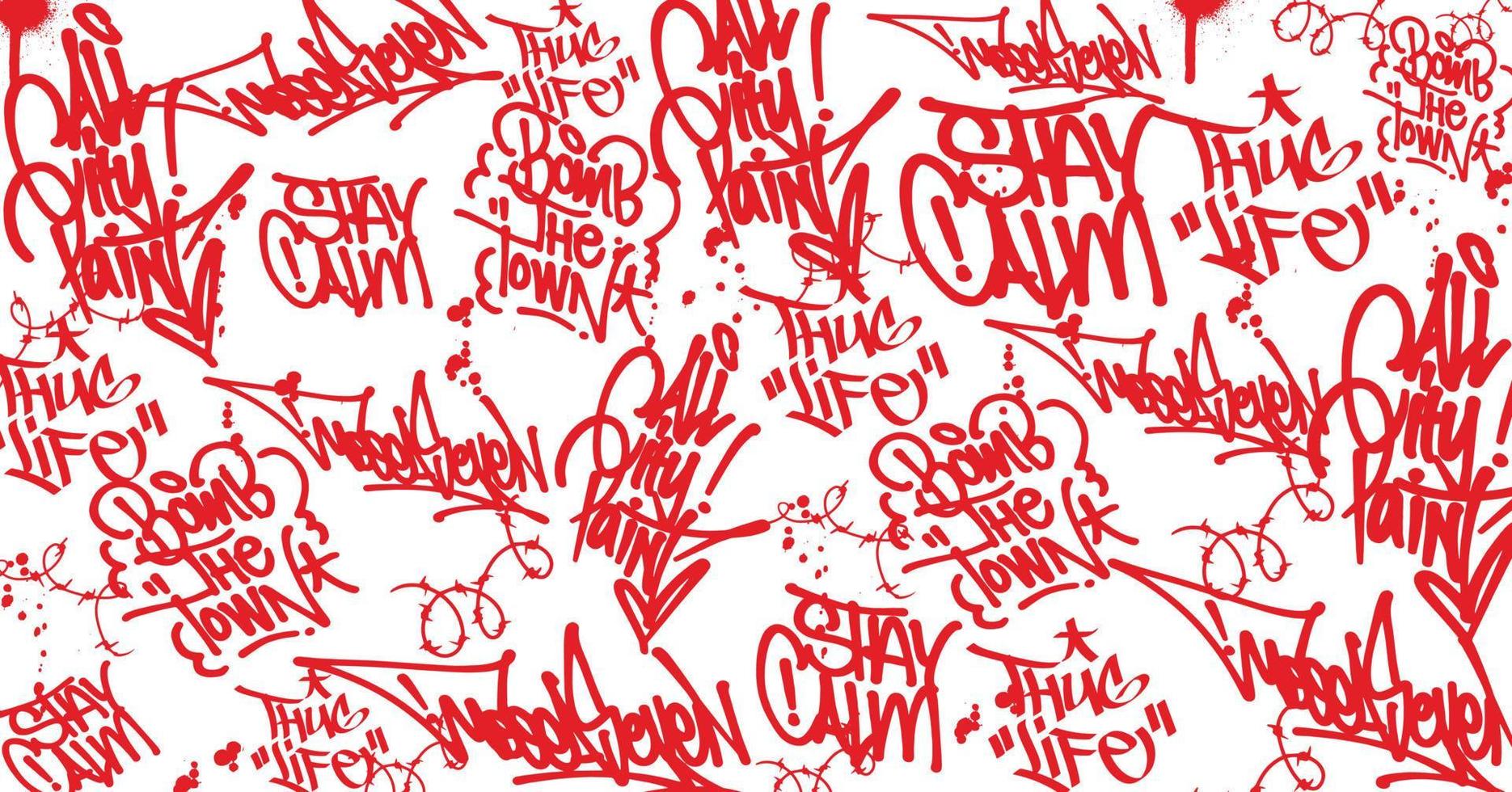The image features a white surface densely covered in red writing, mimicking a graffiti style. Various phrases, primarily "Thug Life," "Stay Calm!" with an exclamation mark, "Bomb the Town," and "All City Paint," repeat frequently across the surface in a range of fonts, including cursive and more elaborate graffiti-inspired scripts. Scattered barbed wire illustrations and splatter decorations accentuate the chaotic and layered composition, creating the appearance of words overlaid upon one another. The repeated phrases are interspersed throughout the image, with notable placements such as "Thug Life" often paired with small stars or barbed wire embellishments. The entire canvas is unified by the consistent use of a deep red color, giving the piece a cohesive yet dynamic look.